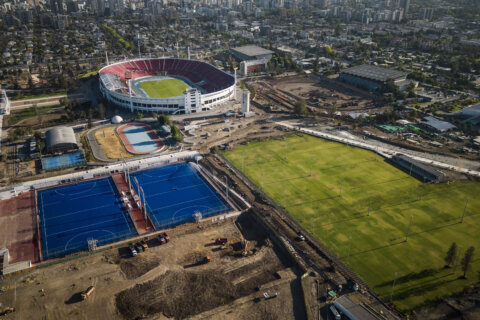The image is an aerial shot of a sprawling sports complex adjacent to a cityscape that transitions from smaller homes to towering skyscrapers. Central to the complex is a football stadium, featuring a grass field and red seating arranged in a single deck. Directly behind it lies a subdivision of small homes. Surrounding the stadium are various sports facilities: two blue basketball courts side-by-side, a smaller track with an orange track surface and a blue center, and nearby, a pair of blue tennis courts. To the bottom right of the stadium, there are multiple grass fields and a couple of indoor sporting facilities. The bottom left corner of the complex shows an active construction site, hinting at future expansions. The overall layout appears somewhat surreal, perhaps due to digital rendering, but it emphasizes diverse sports amenities within a compact area.